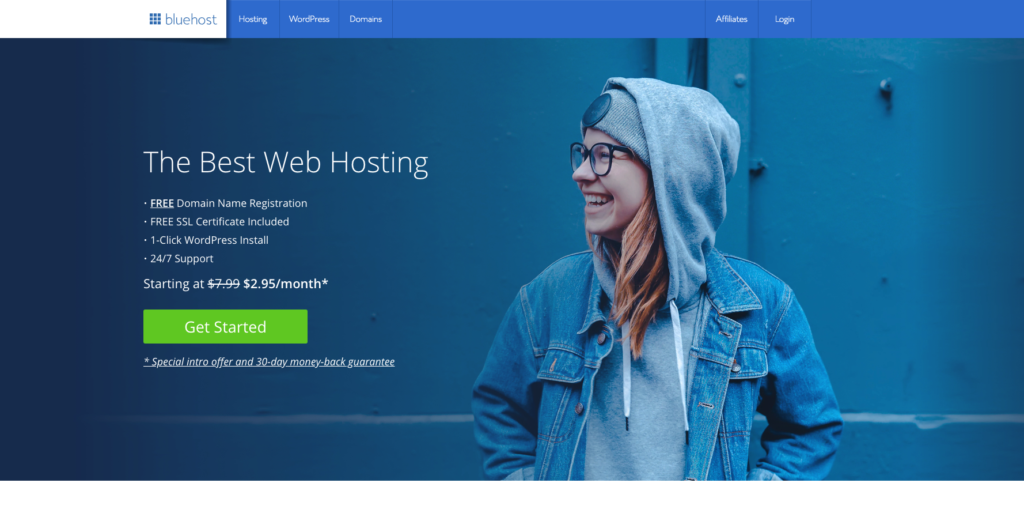The image features a young woman with reddish hair, wearing a layered outfit that includes a hooded sweatshirt underneath an open denim jacket. The jacket has two strings hanging down, and it appears that she has her hands tucked into its pockets. She is also wearing a hat beneath the hood, which is adorned with a prominent black circle on the front. The woman is smiling and looking to her right, with glasses perched on her nose.

Beside her, several promotional texts are displayed, suggesting web hosting services. The text reads, "The best web hosting," followed by highlights such as "Free domain name registration," "55 L certificate included," "One-click WordPress install," and "24/7 support." The initial price of $7.99 per month is crossed out, showing a discounted rate of $2.95 per month. A large green button labeled "Get Started" emphasizes the offer, stating "Special intro offer" and a "30-day money-back guarantee."

Above this, the text "This is hosted by Bluehost" is prominently displayed in blue, accompanied by a box with a grid of nine dots. Additional texts in the box include "Hosting," "WordPress," "Domain," and options like "Affirm" and "Log In."